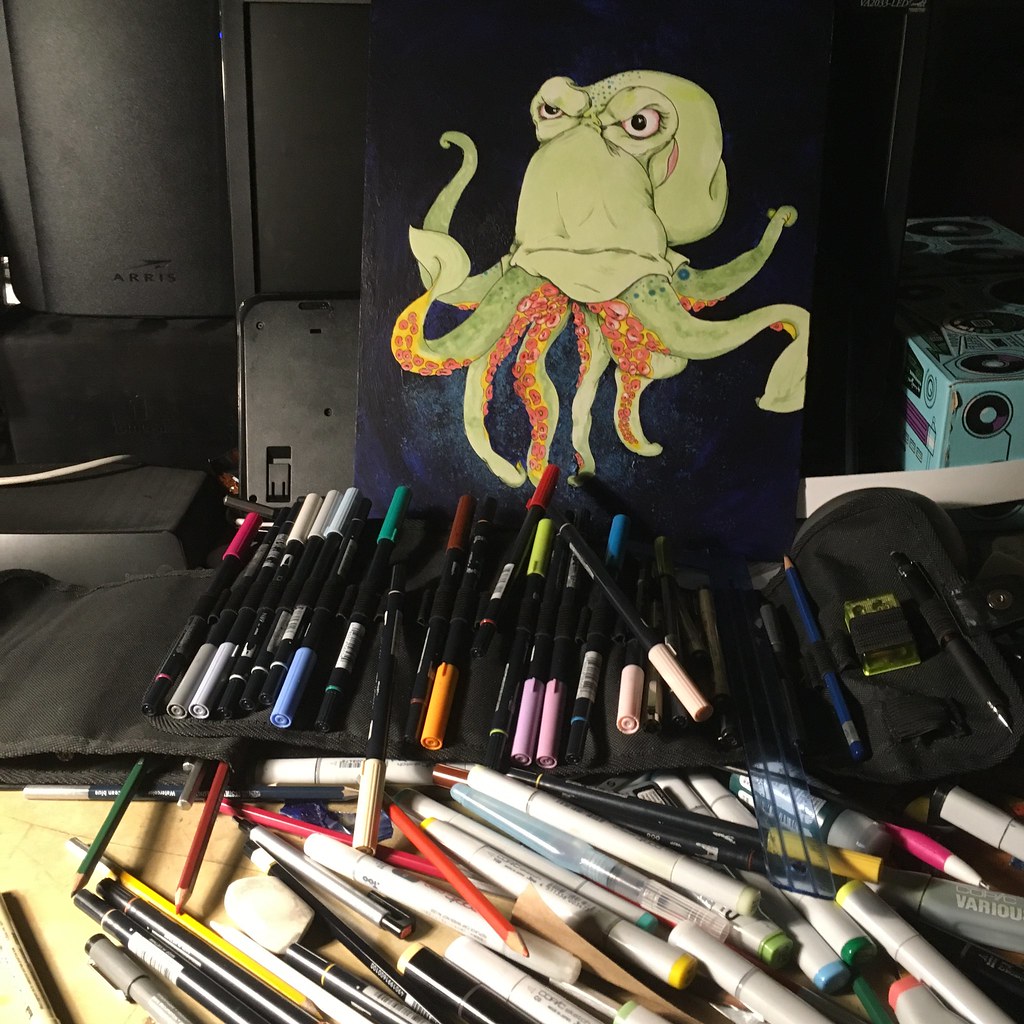The image features an art scene with numerous colorful art supplies arranged predominantly in the lower half of the image. There is an assortment of markers, some of which are identified as Copic markers, alongside colored pencils. Many of these tools are neatly stored in a black pouch or sleeve, while others are scattered across the surface. The markers and pencils come in a variety of vibrant colors, including red, brown, green, yellow, blue, pink, maroon, orange, and white. Additionally, there's an eraser amidst the supplies.

Above these supplies, there is a striking painting of a green octopus on a canvas. The octopus has a grouchy expression, with its eyes looking fierce. The tentacles of the octopus feature orange or red suckers, and the background of the painting is predominantly bluish. The artwork appears to be propped up by a black device, possibly a screen stand. In the upper parts of the image, there is a black device, identified as a modem or router, with the label R-A-R-R-I-S, visible in the upper left-hand corner. Contributing further to the blue tones in the image, a turquoise box can be seen on the right-hand side. The table surface under the art supplies seems to have a yellowish hue.